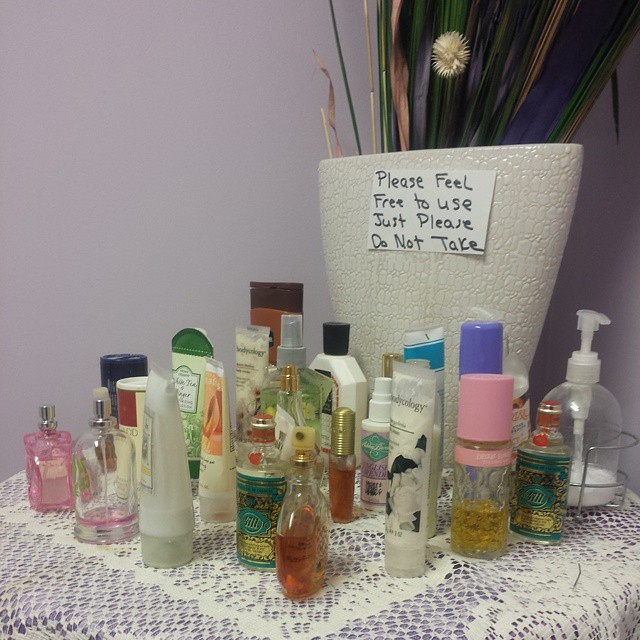This poorly lit, square, full-color indoor photograph showcases a diagonally positioned table draped with a lace tablecloth and a lace table mat, adorned in a purple and white color scheme. The backdrop features a lavender wall that sets a serene atmosphere. At the rear left of the table stands a striking white, wide vase with a distinct textured, bubbly or crocodile skin look, housing green and brown stalks alongside a single white flower. Taped to the vase is a handwritten note on a white card reading, “Please feel free to use, just please do not take.” The table itself is covered with approximately 20 various personal care products, including perfumes, lotions, skin creams, and body wash, some with their caps off and others still on, all arranged neatly in several rows.